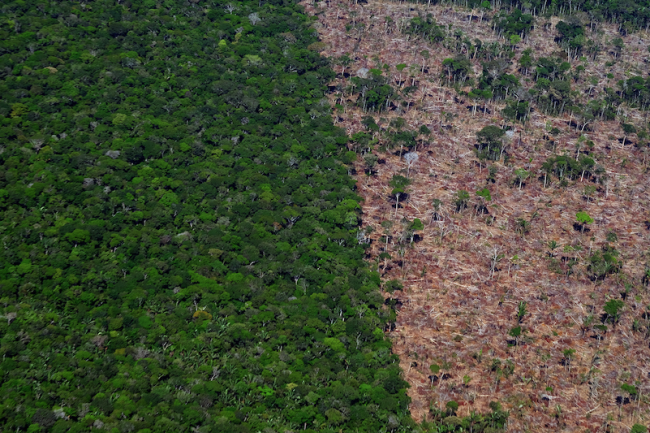This aerial photograph vividly captures a stark contrast between two distinct halves of a forested landscape. The left side of the image is densely populated with lush, dark green treetops, likely a part of the Amazon rainforest, showcasing various shades of green that blend seamlessly with some visible tree formations. In juxtaposition, the right side of the photograph reveals a desolate area marked by deforestation, featuring predominantly bare soil with sporadic, isolated trees. The division between these two areas occurs diagonally from the top left to the bottom right, creating a natural yet distinct boundary. The barren region on the right includes mottled patches of pink, white, and yellow, giving an impression of exposed earth and possibly suggestive of remnants of vegetation. This striking image highlights the impact of deforestation, with the once-thriving forest reduced to scattered outcroppings and pockmarked areas amidst a vast expanse of cleared land.